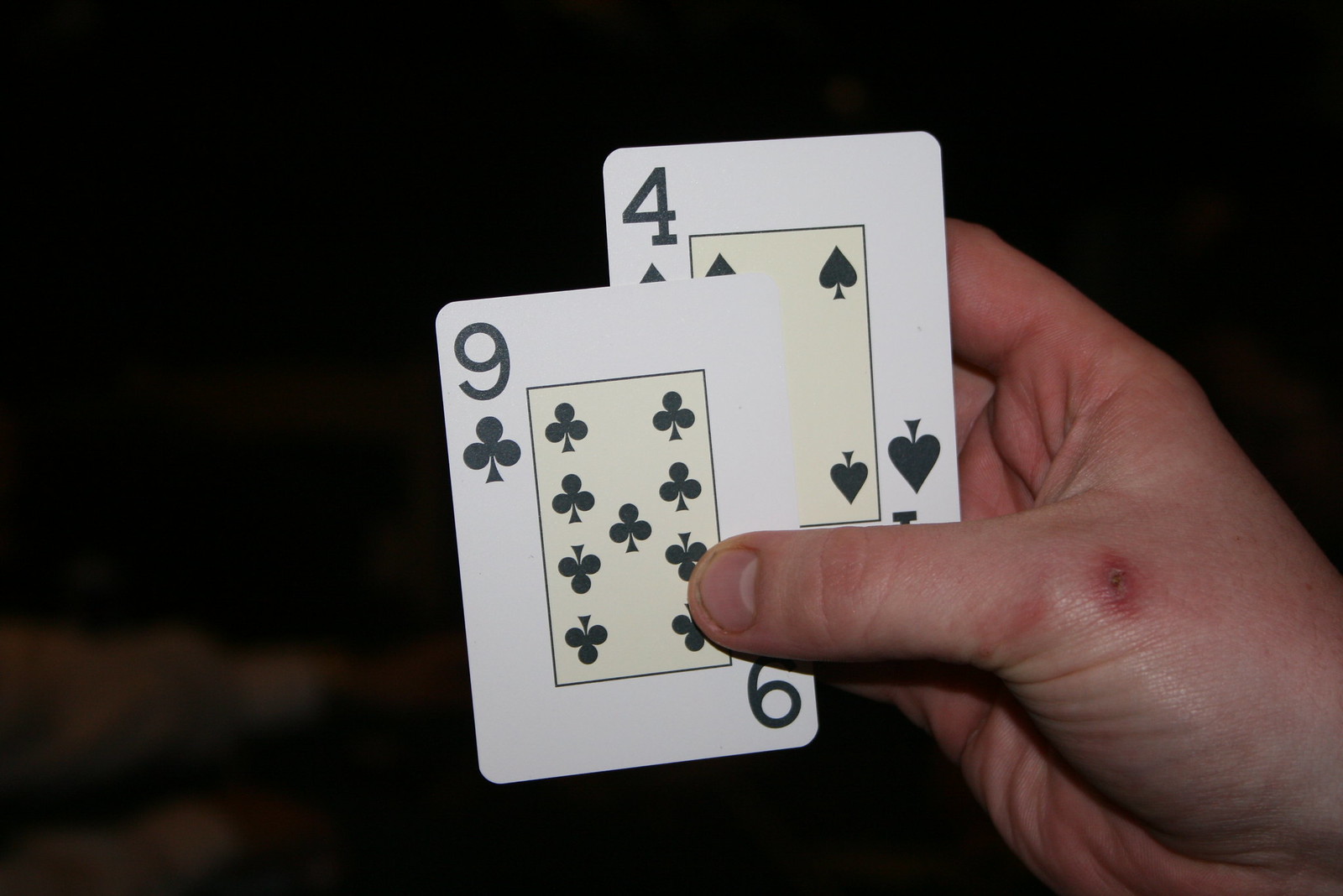A close-up image captures a man's right hand holding two playing cards: the Four of Spades in front of the Nine of Clubs. His hand shows an injury at the base of the thumb, which has formed a scab and appears to be healing well. The cards are held up against an indistinct background, where the bottom left corner reveals the forearms and hands of another person, donned in a long-sleeved white shirt. This could suggest that the setting is informal, likely a home game among friends rather than a casino, given the visible arm of another player and the casual vibe conveyed by the photograph.